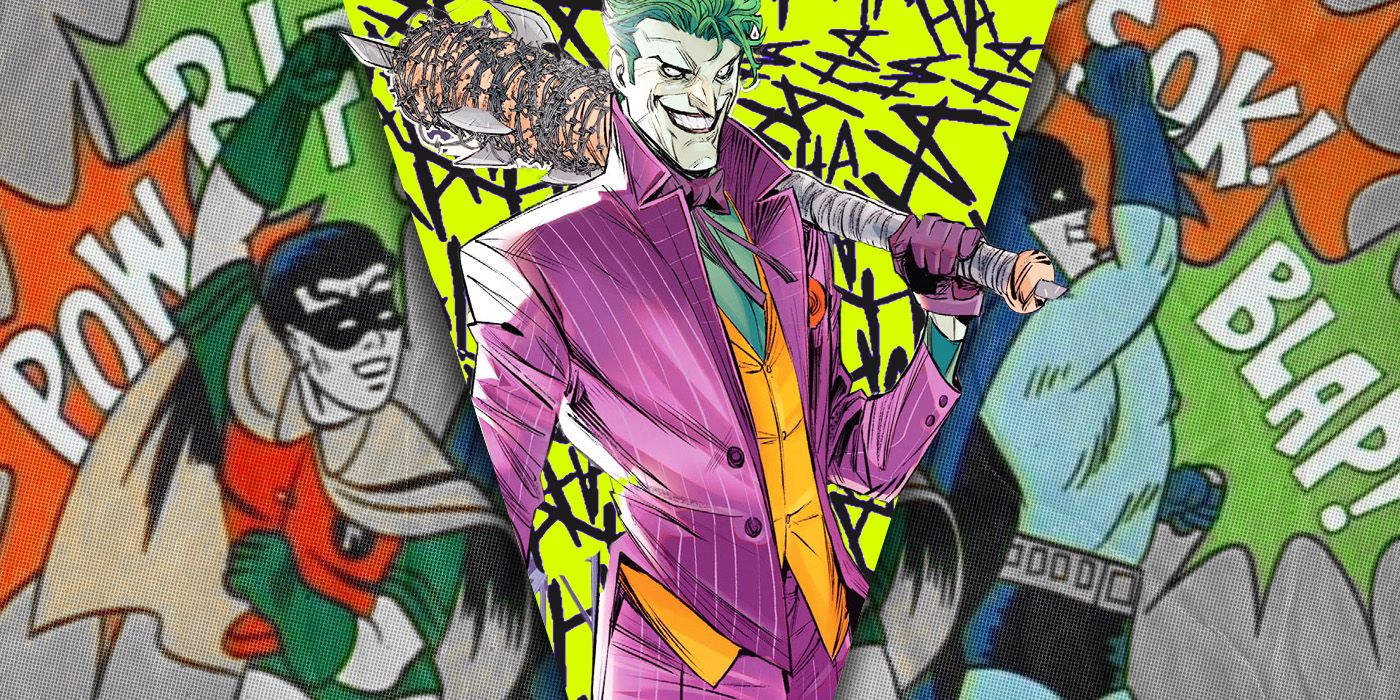The image is a vivid collage of various comic book illustrations featuring iconic characters from the Batman series. On the left side, an older depiction of Robin is shown, characterized by his black hair, white-gray skin, and a black mask covering his eyes. He is outfitted in a red vest over a green tunic, green gloves, light brown cape, and has both fists clenched, with the left lowered and the right raised above his head. Behind him, explosive sound effect shapes in red and green, outlined in black, display the words "POW," "BLP," and "BIFF" in bold, white text.

In stark contrast, the center of the image showcases a modern, sophisticated rendition of the Joker. He sports a nefarious grin and his traditional purple suit with white pinstripes, paired with an orange vest and a blue shirt underneath. His vibrant green hair and menacingly exaggerated facial features set him apart from the other characters. The Joker wields a brutal, Negan-like baseball bat wrapped in chains, blades, and metal wire, emphasizing his dangerous persona. The background behind him is a chaotic yellow, littered with the word "HA HA" in black, echoing his maniacal laughter.

On the far right, an old-school Batman is depicted in his light blue and black suit. He wears a gray or silver utility belt, his iconic bat mask, and blue gloves adorned with long spikes. Emphasizing his dynamic presence, text bubbles in red and green with the words "SOCK!" and "BLAP!" are placed behind him, outlined in black with sharp, splatter-like edges.

The blend of nostalgic and modern artistic styles throughout the piece highlights the timelessness and evolving nature of these legendary characters.